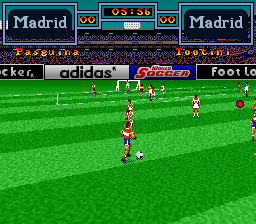This is a detailed screenshot of a soccer field from a computer game. The field is visually striking with thick alternating stripes of green and darker green. In the upper right and left-hand corners, there are black squares outlined in light blue, each displaying the word "Madrid" in white text. Flanking these squares are two additional blue squares, each featuring orange double zeros. Positioned centrally and slightly higher between these squares is a prominent black rectangle with vibrant orange and yellow numbers displaying "05," alongside a vertical line that reads "56."

On the field, soccer players are visible, though they appear more as abstract forms characterized by vivid splashes of yellow, red, and white, with one player positioned conspicuously in the center. The overall scene captures the dynamic and vibrant atmosphere of a digital soccer game.